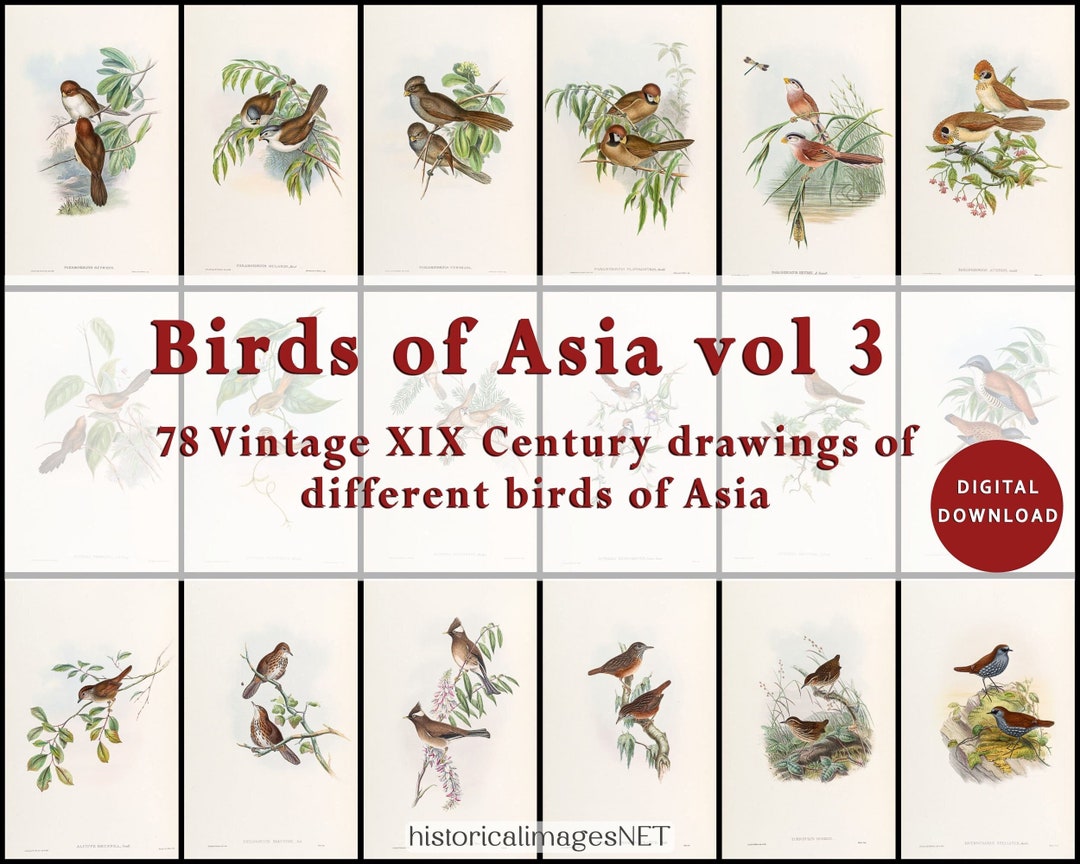The image is an up-close sectional of what appears to be a book cover titled "Birds of Asia, Volume 3, 78 Vintage XIX Century Drawings of Different Birds of Asia." This title is centrally placed in maroon text. To the right, there is a label that says "Digital Download" in white text within a maroon circle. At the bottom center, the text reads "Historical Images Net."

The poster is divided into three horizontal sections. The top section showcases six images, each featuring two brownish birds with white plumage, perched on branches or tree limbs. These birds, while of the same type in each image, are captured looking in different directions—some towards each other, some away. The illustrations also incorporate natural elements such as green foliage, pink buds, and even a dragonfly.

The middle section is dominated by the main title which partially covers the second row of bird images, causing them to appear out of focus and grayed out.

The bottom section mirrors the top, displaying another set of six similar bird images with the birds again looking in various directions. Each bird illustration is still not labeled, and the tiny text present on the images remains unreadable. The background of the poster is white, while the bird images are set against an off-white backdrop.